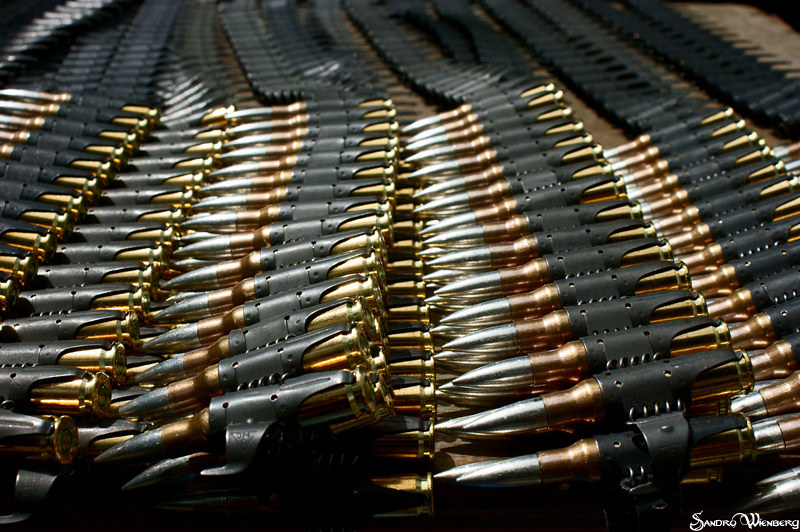In this photograph, the scene is dominated by thousands of bullets meticulously arranged in black bullet belts, creating massive stacks that fill the entire frame. The bullets feature striking silver tips with copper-colored bodies, lending a sharp contrast against the dark belts. The bullets are organized in four visible rows of vertical columns, with numerous additional belts layered beneath them. The image is densely packed with these ammunition belts, occupying the entirety of the visible space. The setting appears to be indoors, possibly in an ammunition warehouse. Colors in the photograph include black, gold, silver, gray, and tan, enhancing the industrial and austere feel of the scene. A watermark at the bottom of the image reads "Sandra Winberg," but no other text is present.